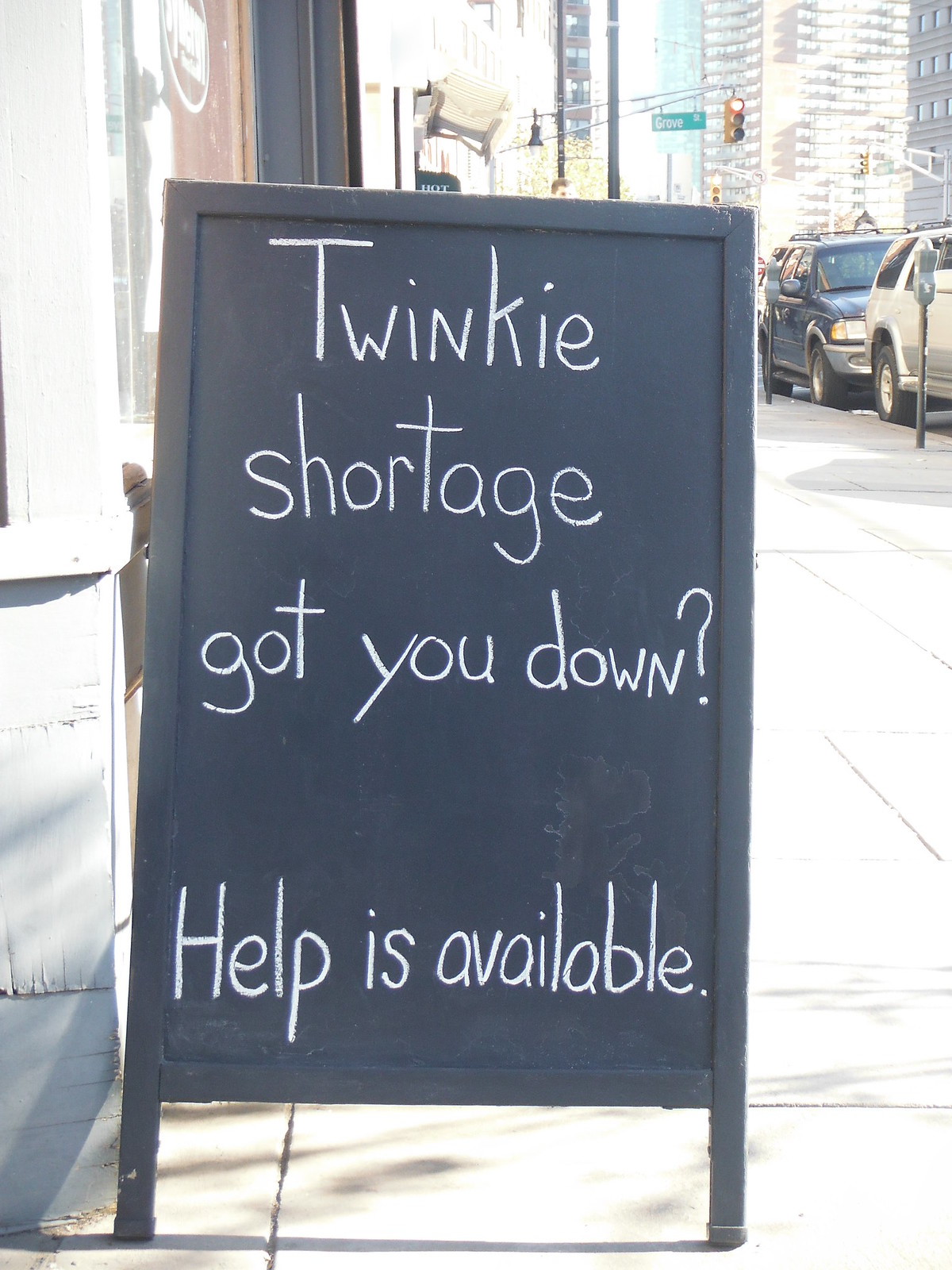The photograph depicts a bright city sidewalk scene taken during the daytime. The image, in portrait orientation, showcases a black, fold-out chalkboard sign with white chalk writing prominently displayed against a gray stone building on the left. The sidewalk appears bright due to the intense lighting, and a brown door is slightly visible behind the sign. The black sign, with two legs visible and presumably double-sided, features an inscription in three rows of text: "Twinkie Shortage got you down? Help is available," with only the 'T' and 'H' capitalized. To the right of the sign, the street has parked vehicles—a black SUV and a gray SUV, partially seen—alongside a parking meter. In the background, tall skyscrapers dominate the cityscape, and red traffic lights and a street name sign add urban context. The overall brightness makes the image somewhat washed out, focusing attention mainly on the chalkboard sign.